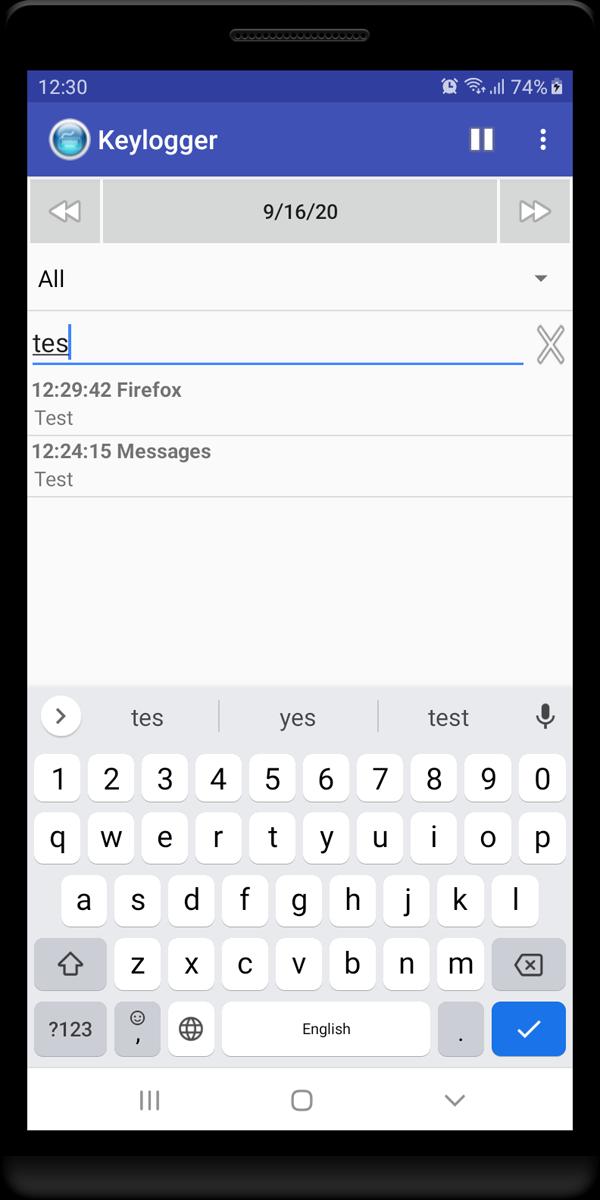This image displays a smartphone screen with a battery level at 74% and the time shown as 12:30. The device appears to be manufactured by Keylogger. The interface features a turquoise circle icon, set against an initially gray bar that also shows the date as 09-16-20. Two directional arrows, one pointing left and one right, are visible within a lighter gray bar. 

The text "TES" (typed as T-E-S) is entered, accompanied by a large X next to a blue line. Further down the screen, timestamps such as "12-29-42 Foxfire" and "12-20-4-15 messages" are visible, indicating some form of ongoing test. 

A virtual keyboard occupies the bottom portion of the screen, and a blue checkbox is ticked on the right side. Below the text entry field, there are several icons, including three horizontal lines, a box, and a downward-pointing dropdown arrow. A larger menu button featuring three circles and a vertical line is positioned at the top of the screen.